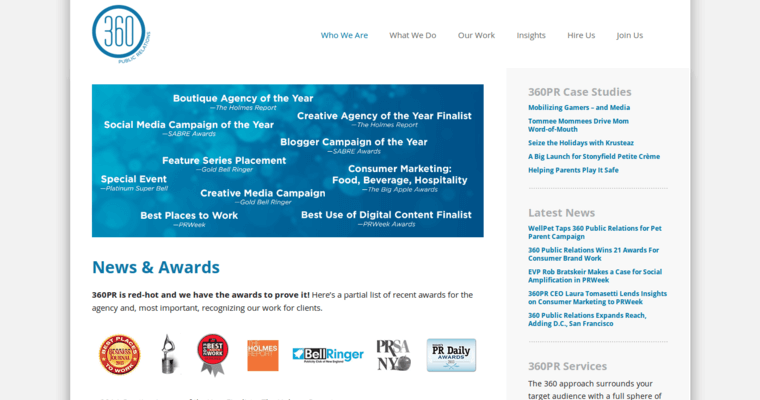**Detailed Caption:**

This image is a screenshot of a webpage belonging to 360 PR, characterized by a predominantly white background. In the upper left corner, the 360 logo is enclosed within a blue circle, accompanied by the text "Public Relations" on the outer edges. Positioned at the top right are navigational menu headings including "Who We Are," "What We Do," "Our Work," "Insights," "Hire Us," and "Join Us."

Directly below the navigation bar lies a large rectangular section, stylized with a blue marble shade and adorned with white text. This section highlights various accolades such as "Boutique Agency of the Year," "Creative Agency of the Year Finalist," "Social Media Campaign of the Year," "Blogger Campaign of the Year," "Feature Series Placement," "Consumer Marketing," "Food, Beverage, Hospitality," "Special Event," "Creative Media Campaign," "Best Places to Work," and "Best Use of Digital Content Finalist." The names of the awarding publications are listed in a smaller font beneath these accolades.

Further down, a header reads "News and Awards," followed by the statement "360 PR is red hot, and we have the awards to prove it. Here's a partial list of recent awards for the agency, and most importantly, recognizing our work for clients." This is succeeded by a list of various agencies, each represented with icons.

On the right side of the webpage, a section titled "360 PR Case Studies" showcases different campaigns such as "Mobilizing Gamers," "Seize the Holidays with Crustace," "A Big Launch for Stonyfield Petite Crame," and "Helping Parents Play It Safe." Below this section, "Latest News" is displayed with five accompanying headlines.

Overall, the page exudes a clean, professional look with ample white space, focusing on the achievements and offerings of 360 PR.